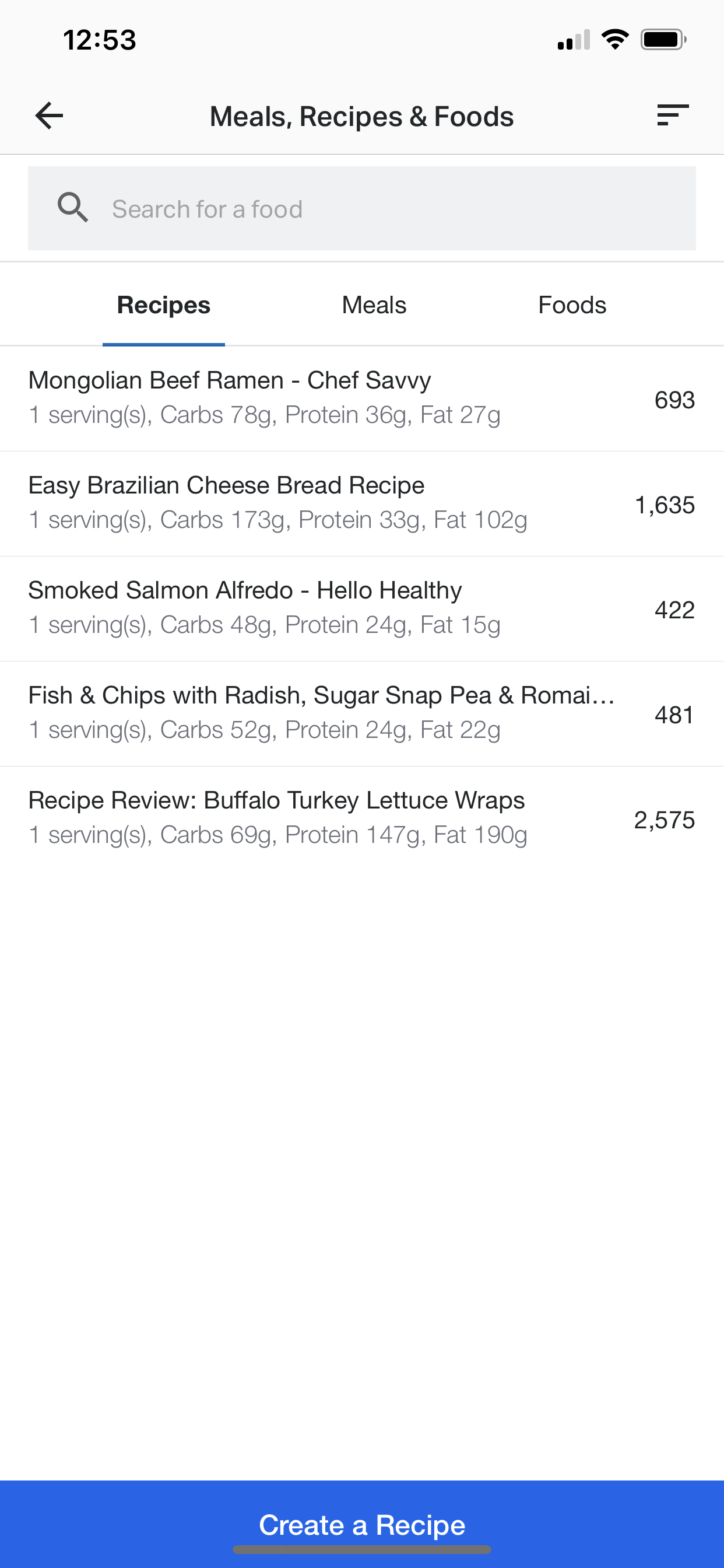**Detailed Caption:**

This screenshot depicts a mobile application interface focused on meals, recipes, and foods. The interface features a light gray header containing a left-pointing gray arrow. Adjacent to the arrow is the title "Meals, Recipes, and Foods" in clear text. On the far right of the header are three horizontal gray lines of increasing height stacked vertically.

Beneath the header, the primary background of the page is white. At the very top, a light gray search bar is centered, with a dark gray magnifying glass icon on the left and the placeholder text "Search for a Food" in light gray.

Below the search bar, a thin light gray line divides it from the content section. This section begins with three segmented options: "Recipes" in bold, blue-underlined text (indicating it is currently selected), "Meals" in gray, and "Foods" also in gray, each separated by thin gray lines.

The selected "Recipes" section displays a list of individual recipes with detailed nutritional information. Each entry is separated by thin light gray lines and includes the following:

1. **Mongolian Beef Ramen, Chef Savvy**
   - **Servings:** 1
   - **Carbs:** 78 grams
   - **Protein:** 36 grams
   - **Fat:** 27 grams
   - **Number:** 693
   
2. **Easy Brazilian Cheesy Bread Recipe**
   - **Servings:** 1
   - **Carbs:** 173 grams
   - **Protein:** 33 grams
   - **Fat:** 102 grams
   - **Number:** 1635
   
3. **Smoked Salmon Alfredo, Hello Healthy**
   - **Servings:** 1
   - **Carbs:** 48 grams
   - **Protein:** 24 grams
   - **Fat:** 15 grams
   - **Number:** 422
   
4. **Fish and Chips with Radish, Sugar Snap Pea, and Romaine**
   - **Servings:** 1
   - **Carbs:** 52 grams
   - **Protein:** 24 grams
   - **Fat:** 22 grams
   - **Number:** 481
   
5. **Recipe Review, Buffalo Turkey Lettuce Wraps**
   - **Servings:** 1
   - **Carbs:** 69 grams
   - **Protein:** 147 grams
   - **Fat:** 190 grams
   - **Number:** 2575

Each recipe item includes the dish title in a slightly darker gray text, nutritional details in lighter gray text, and a numerical identifier to the right.